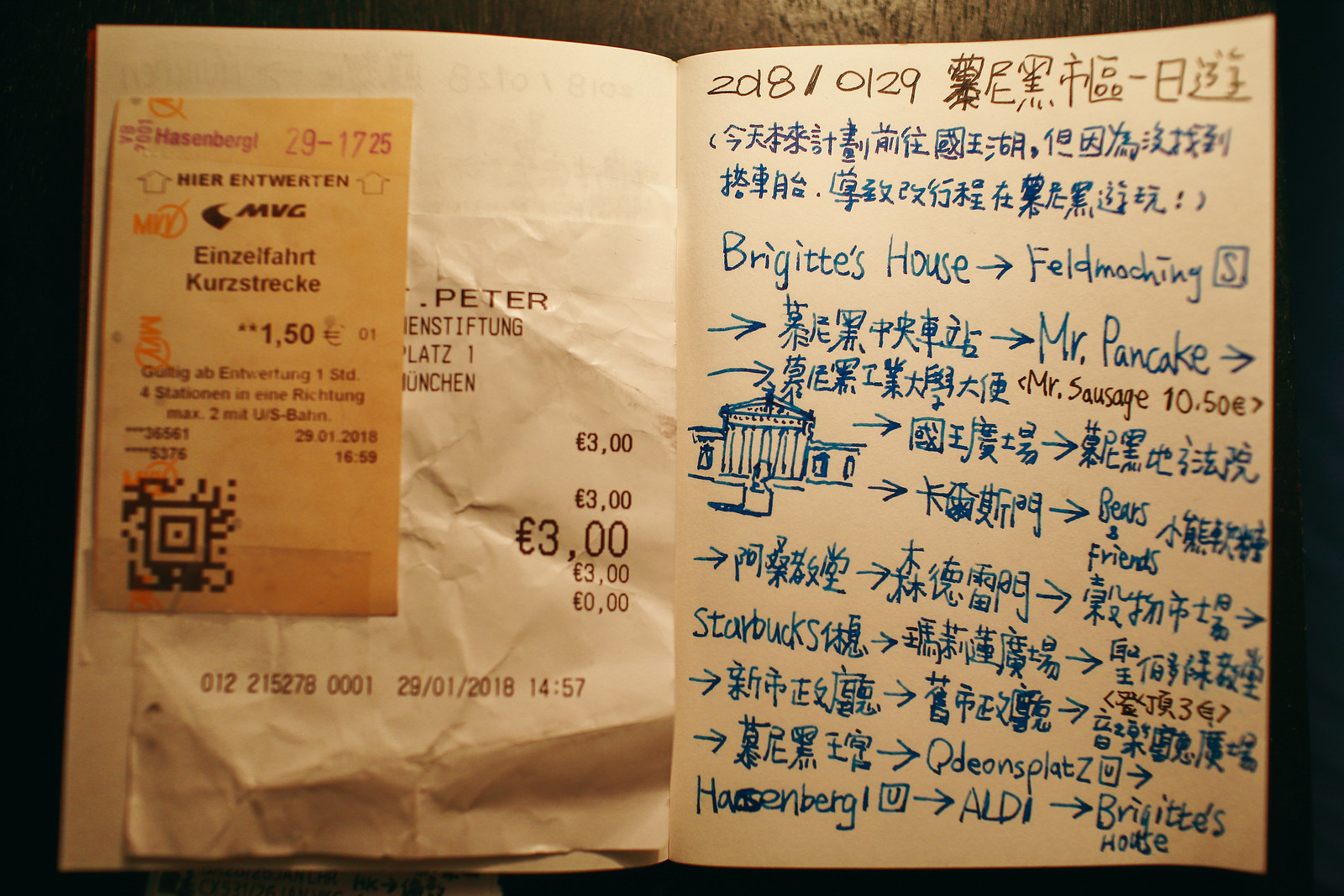The image features what appears to be a diary or notebook open on white paper. On the left side, there are two receipts. One, written in a foreign language, is small, dark-colored, and has a yellow tint. Beneath it lies a larger, white receipt. On the right page, a mix of foreign characters and English text is present. At the top, the text reads "2018/0129," followed by "Bridget's house" with an arrow pointing to "Feldmocking." Further arrows guide the eye to additional foreign characters, interspersed with several notable English phrases: "Mr. Pancake," "Mr. Sausage," illustrated with a sketch of a building. Additionally, "Bears and Friends," "Starbucks," "Odin's Plots," and "Aldi" are listed. The sequence concludes back at "Bridget's house."